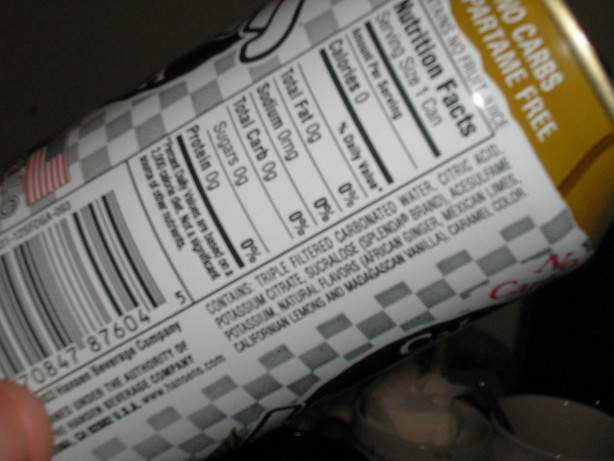In this detailed photograph, a person's thumb is prominently visible as they hold a can of a beverage close to the camera. The beverage can is white with a gray checkered pattern, accented by a gold ring around the top. Clearly legible is a white nutrition facts label in black font, stating that the serving size is one can, containing no calories, fat, sodium, carbohydrates, sugars, or protein. A barcode is also visible on the can. The list of ingredients includes triple filtered carbonated water, citric acid, potassium citrate, sucralose, natural flavors, Mexican limes, California lemons, Madagascar vanilla, and caramel color. In the blurred background, there is a bowl with a spoon inside it and another bowl with a napkin resting in it, adding a homey kitchen context to the scene.